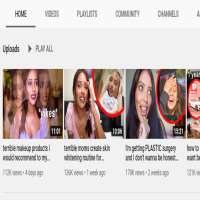This image is a screenshot of a YouTube search page with the "Home" tab selected, indicating that this is the main browsing section. The tabs for "Videos," "Playlists," "Communities," and "Channels" are also visible, suggesting different categories for content browsing on the channel. Below the tabs, there are options labeled "Upload" and "Play All." 

The page lists a few video thumbnails with brief descriptions and timestamps. The first video, uploaded approximately four hours ago, is titled "Terrible Makeup Products" and features a girl wearing poorly applied makeup. The video's title seems to cut off, suggesting it might finish with "to Their Enemies," and has a duration of around 11 minutes.

To the right of this video is another thumbnail with the partially visible title "Terrible Something Cream Skin," which appears blurry. The video, which was uploaded about seven weeks ago, also features the same girl and has a duration of approximately 12 minutes.

The third video listed is titled "I'm getting plastic surgery and I don't want to be honest." It also features the same girl, runs for about 13 minutes, and completes the set of videos on this YouTube search page.